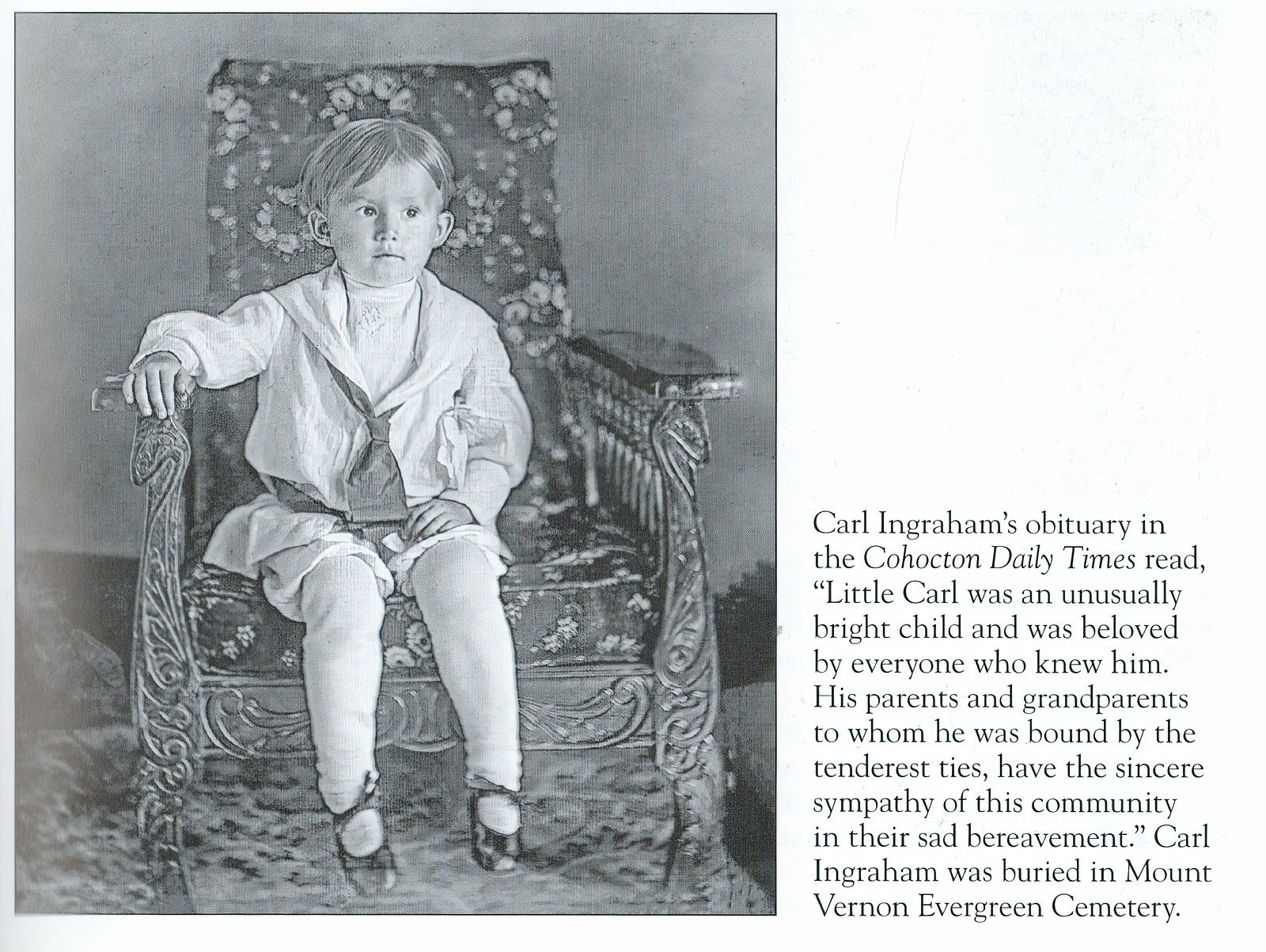This wide rectangular image presents a poignant scene, capturing a black-and-white photograph on the left against a very light gray background, with a caption to the right. The photograph, taller than it is wide, portrays a young child, no more than a year old, seated on an ornately designed chair. The chair features elaborate wooden armrests and legs, along with a floral velvet-patterned cushion. The child, whose feet do not touch the ground, is dressed in a loose, sailor-style outfit complete with a black tie and shorts, black ballet flats, and stockings. Their short hair is neatly parted in the middle, and their right hand rests on the chair's armrest.

Adjacent to this evocative photo is a block of black text on a white background, reading: "Carl Ingraham's obituary in the Cohacktan Daily Times read, 'Little Carl was an unusually bright child and was beloved by everyone who knew him. His parents and grandparents, to whom he was bound by the tenderest ties, have the sincere sympathy of this community in their sad bereavement. Carl Ingraham was buried in Mount Vernon Evergreen Cemetery.'" The professional-quality photograph and the heartfelt obituary together create a touching memorial for Little Carl.